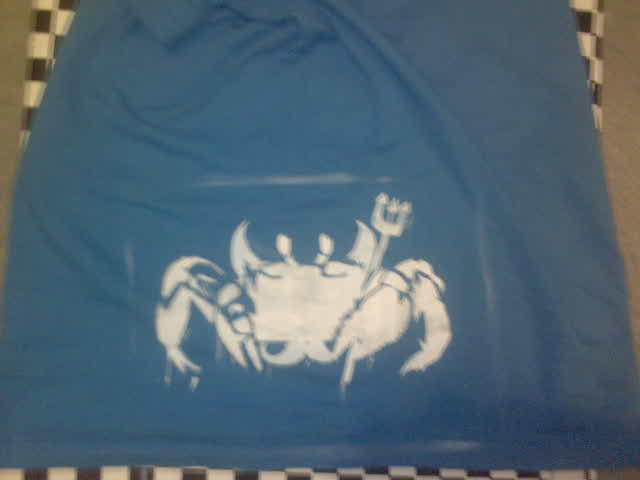The image depicts a section of a chef's apron, featuring a rich royal blue fabric as its primary color. Prominently displayed in the center of the apron is a detailed white graphic of a crab. The crab's left claw is gripping a white pitchfork, which is pointed upwards, adding a whimsical touch to the design. The crab's eyes are visible, protruding slightly from its head, giving it a quirky appearance.

Trimmed along the bottom edge of the apron is a distinct border composed of alternating black and white checks, which also extends up the sides, framing the graphic centrally. The apron appears to be laid out flat on a brown surface, possibly a table or floor. The brown background subtly frames the image, peeking through as thin slivers in the upper corners of the photograph, providing a natural contrast to the vibrant blue of the apron.